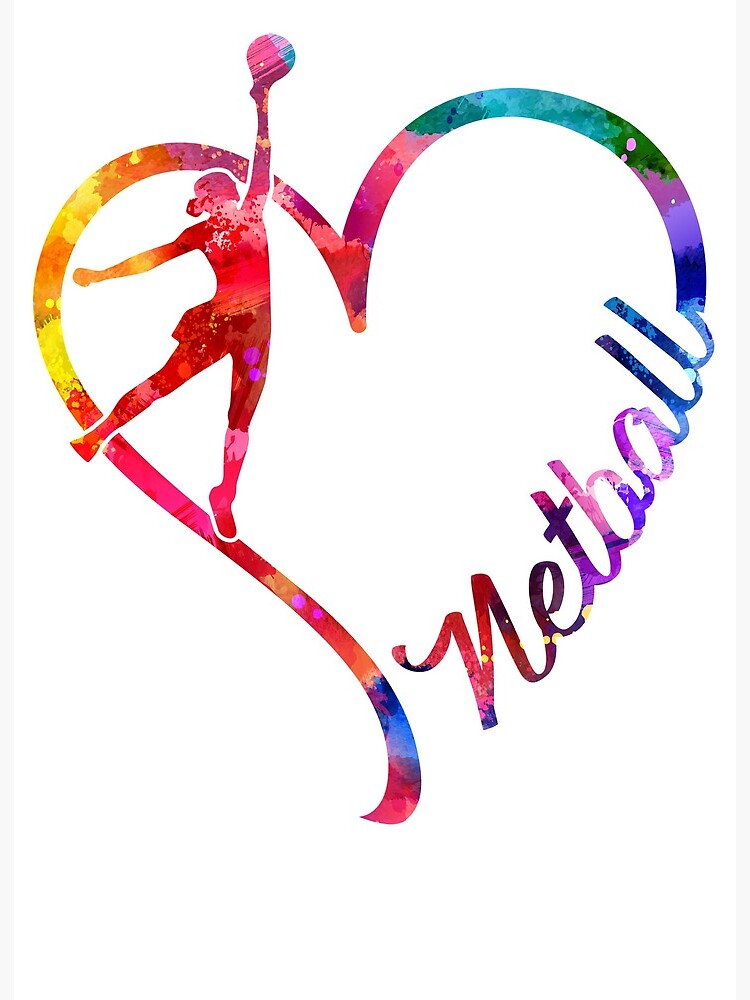In this vibrant and colorful logo on a white background, the word "Netball" is elegantly written in a cursive script, seamlessly integrated into the shape of a heart. This heart is decorated with a beautiful rainbow spectrum, transitioning through shades of red, blue, orange, pink, yellow, green, aqua, and purple, resembling a watercolor effect. The word "Netball" starts at the bottom right of the heart, curves into the first loop, moves downward, and then arcs back up to complete the heart shape. On the left side of the heart, set within the loop, is an image of a female athlete in motion, captured in a dynamic pose. She balances on one foot, her right arm outstretched beyond the heart’s border, and her left arm raised as if she’s about to hit a ball. This figure is illustrated in warm shades of red, orange, pink, and purple, enhancing the sense of movement and energy in the logo. This detailed and colorful depiction beautifully represents the sport of netball.